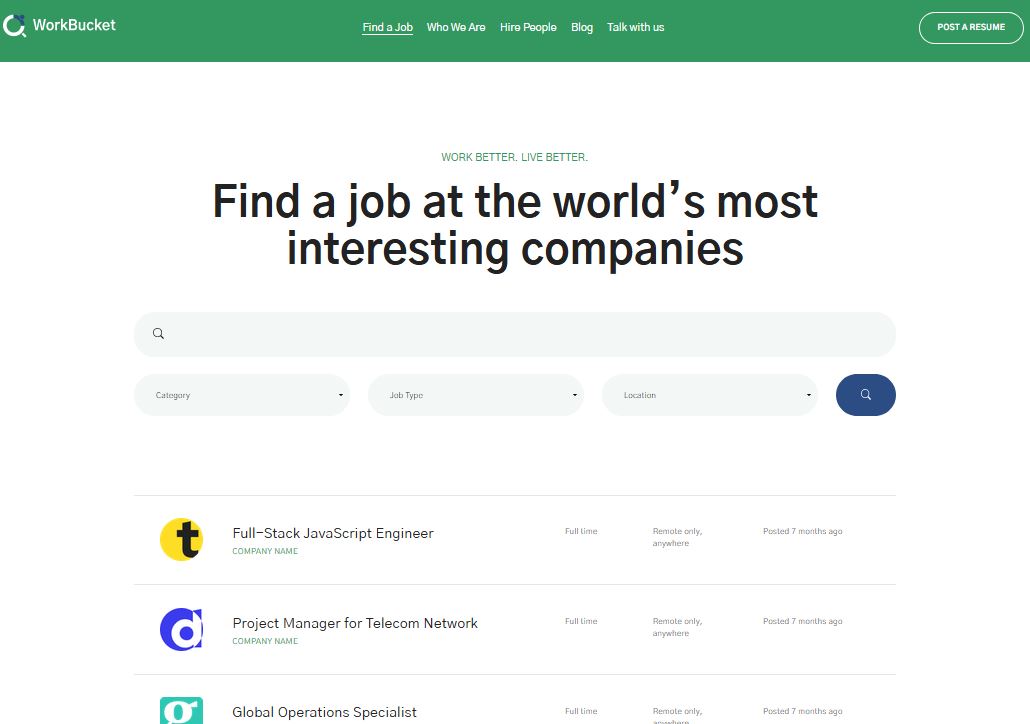This image appears to be a screenshot from a job listing website. The top inch of the image features a dark green border. In the top-left corner of this green border, there is a logo that resembles a sideways 'C' facing upward to the left, with a small blue section in the upper-right that partially closes it off, and a short line descending to the right beneath the 'C'. Adjacent to this logo, white text spells out "Work Bucket".

Below the green border, the background turns white. At the top-center of the white section, in bold black letters, it reads, "WORK BETTER LIVE BETTER". Below this, in even larger bold black text, it says, "Find a job at the world's most interesting companies". 

Central to the image is a large search bar, which extends from approximately two inches from the left edge to about two inches from the right edge. Below this larger bar is a smaller search bar divided into multiple fields: "Category", "Job Type", and "Location". Each field has a designated space, and to the right of these fields is a small search bar featuring a search icon.

Further down the image, a thin gray line spans the width of the page. Below this line, there are job listings aligned vertically. Each listing includes an icon on the left side – the first icon being a yellow circle with a black 'T' in it – followed by the job title (e.g., "Full Stack JavaScript Engineer"), the company's name, the job type (e.g., "Full-time"), the job’s location details (e.g., remote or in-office), and the posting time.

On the far right side of the green border at the top, there are menu options listed in white text: "Find a Job", "Who We Are", "Hire People", "Blog", and "Talk with Us". Additionally, on the right side, there is a green tab with a white border and capitalized white lettering that says "POST RESUME".